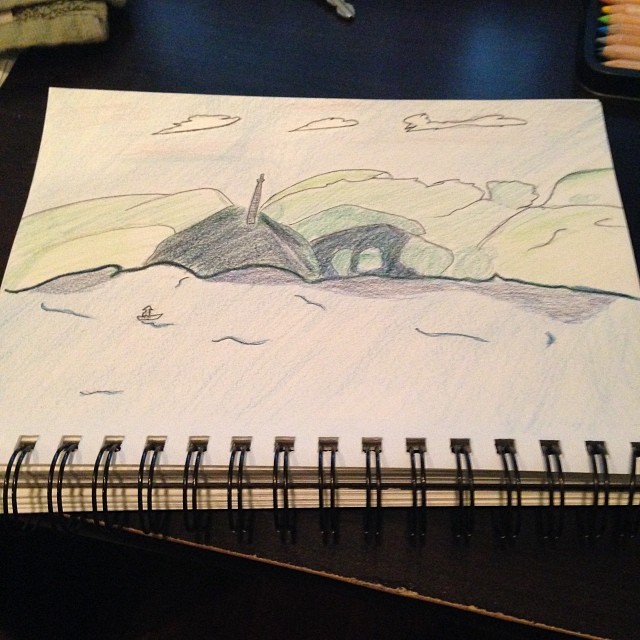A photograph captures a page from a coloring notebook resting on a black table. In the top right corner, the tips of an array of colored pencils can be seen, though most remain out of the frame. The artwork on the page appears juvenile, possibly created by a child, using colored pencils. The scene depicts an ocean covering the bottom half of the page, colored in varying shades of blue, with a small, crudely drawn figure in a boat navigating its waters. Centrally, a landmass extends upward, showcasing green hills and a simple lighthouse perched atop one of them. Above the landscape, a clear sky features three minimalist clouds. Despite its lack of intricate detail, the drawing exudes a charming, innocent quality reflective of a child's imagination.